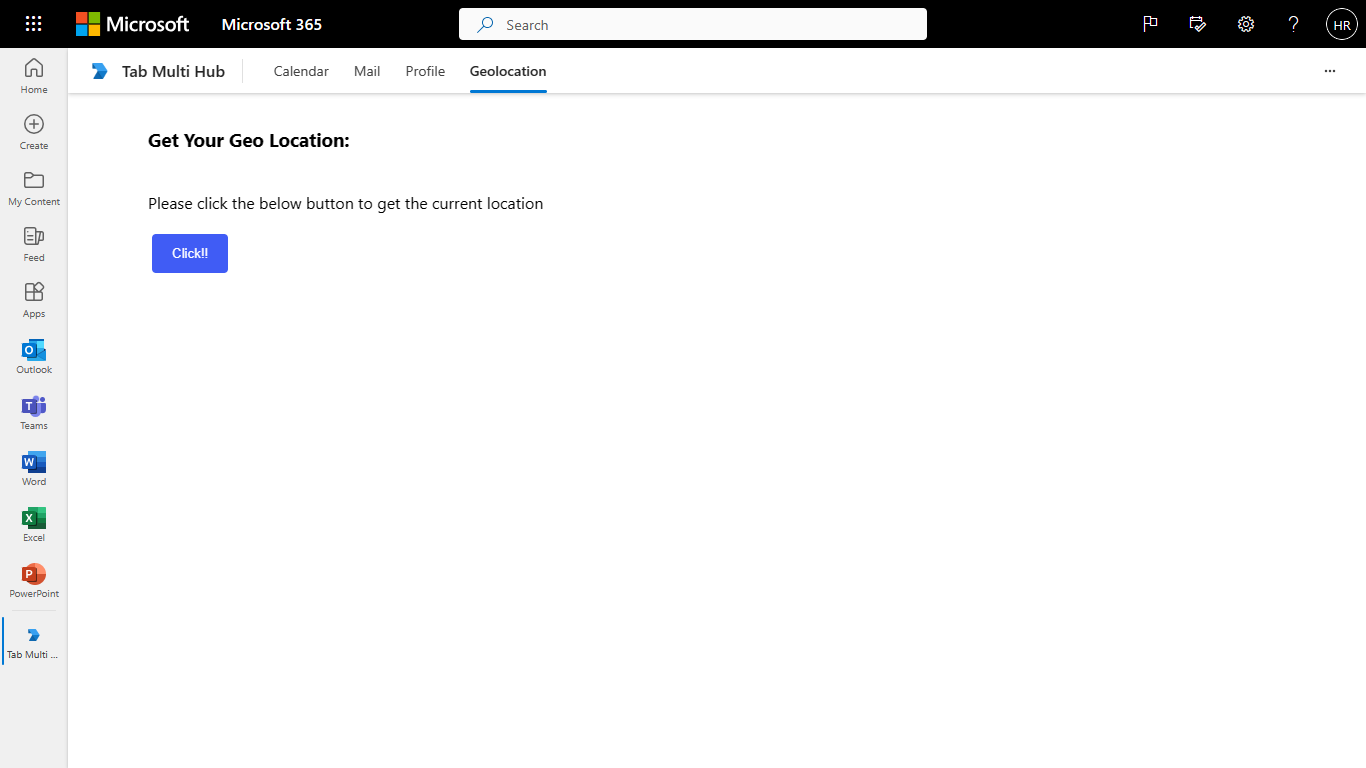### Detailed Caption:

The image is a screenshot of a computer monitor displaying a Microsoft product interface, set in a landscape (horizontal) orientation typical of a laptop or desktop screen. Across the top of the screen is a prominent black bar featuring various icons and text. In the center of this black bar is a white search bar with the placeholder text "Search" and a magnifying glass icon on its left side. To the left of the search bar, the black bar houses a series of icons starting with a 3x3 grid of nine white dots, followed by the Microsoft logo, which is composed of four colored squares (red, green, yellow, and blue) with the text "Microsoft 365" next to it.

On the right side of the black bar, aligned to the right, are several small white icons: a flag, possibly representing a calendar, a settings gear (cog icon), a question mark, and a circular icon featuring the initials "HR," which likely represents the user's initials.

Below the black bar is a white bar underlined with gray, containing tabs labeled "Multi-Hub," "Calendar," "Mail," "Profile," and "Geolocation." The "Geolocation" tab is selected, indicated by a blue underline.

The main body of the screen is predominantly white, with a pale gray column on the left side listing different menu options. While some text isn't legible, the visible options include "Home," "My [Unreadable]," "Feed," "Apps," "Word," "Excel," and "PowerPoint," with some icons displayed in black outline and others in color.

In the central white area below the toolbar, there is a message: "Get your geolocation. Please click the button below to get the current location," accompanied by a blue button labeled "Click!"